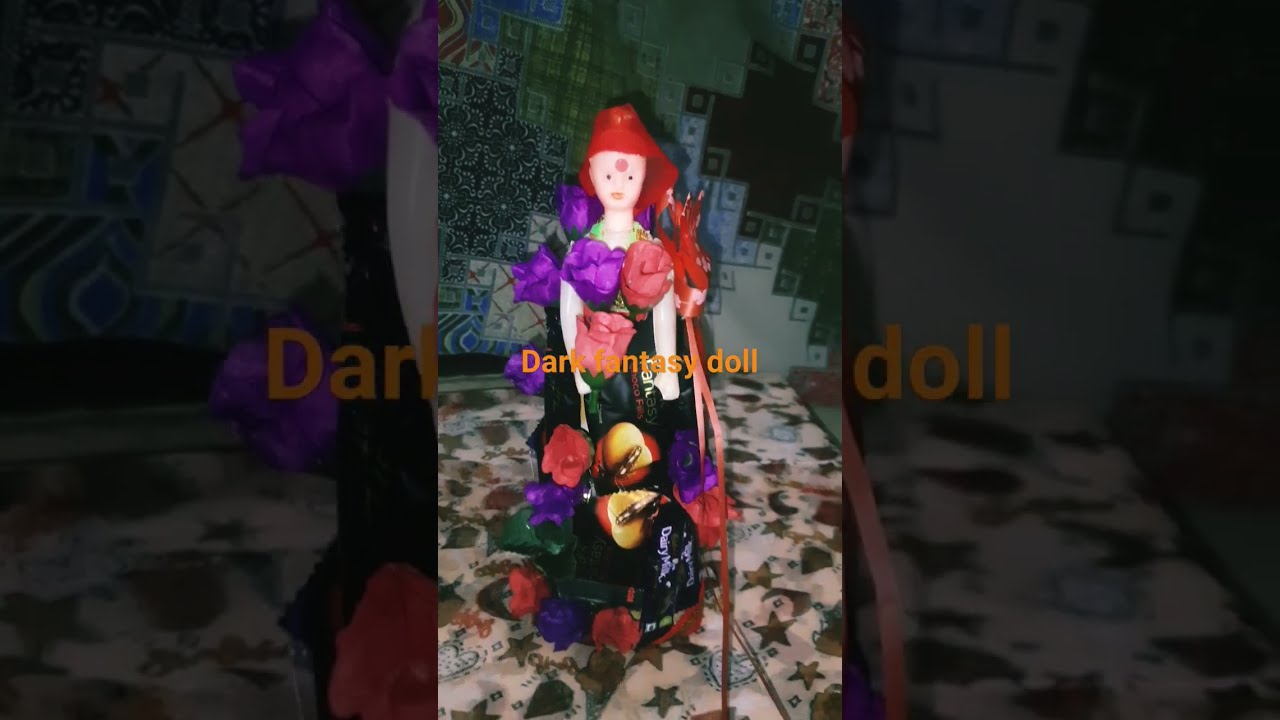The image features a delicate, porcelain-like doll adorned with an intricate floral design in shades of red, pink, purple, and yellow. A small red hat decorates the doll's head, which also has a distinctive dot in the center of the forehead. The doll stands on a vivid, patterned floor that showcases moons and stars. The background is a kaleidoscope of checkered prints and various patterns with fragmented sections that cast a darker tone on the left and right thirds of the image, creating a stark contrast to the brighter center. Dominating the foreground in reflective orange text is the caption "Dark Fantasy Doll," which leaps out against the colorful backdrop. The overall setting is richly detailed with a mix of vibrant colors including red, pink, purple, orange, gold, olive, blue, green, black, white, and gray, adding a fantastical and somewhat whimsical atmosphere to the scene.